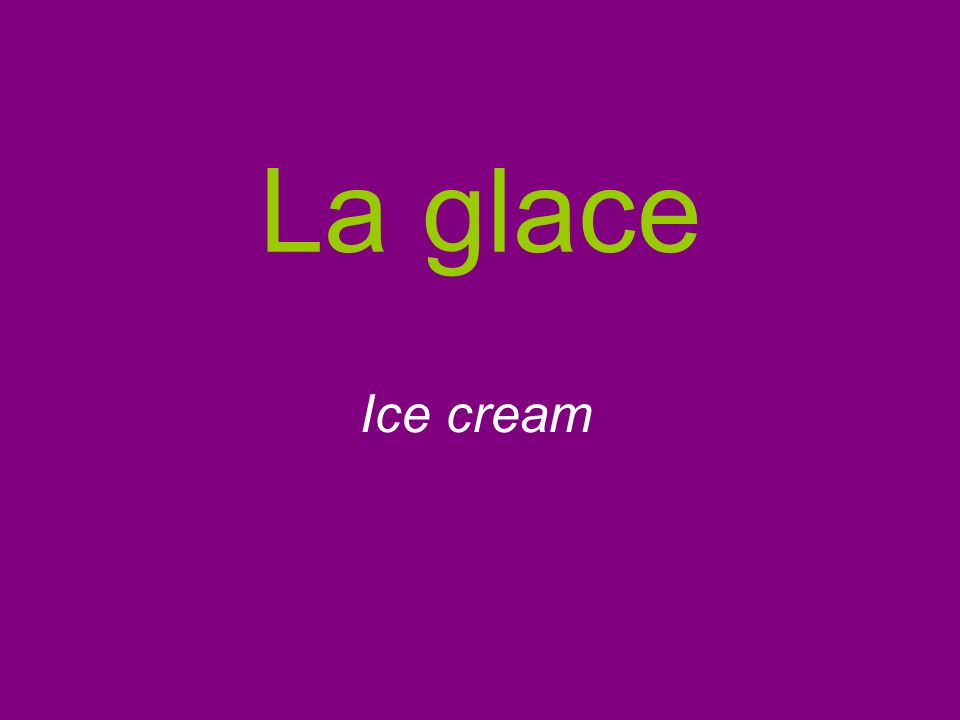On a deep, rectangular purple background with hints of pink, the word "La Glace" is prominently displayed just above the center in a medium green color. The "L" in "La" is capitalized while the "a" is lowercase, and there is a subtle spacing between each letter in "Glace," which is all lowercase. Positioned below "La Glace," but still centered, the word “Ice Cream” is written in smaller, bold white letters with a slight rightward slant. The "I" in "Ice" is capitalized, while the remaining letters are not. This simple yet striking design combines the contrasting colors and fonts to create a visually appealing image.